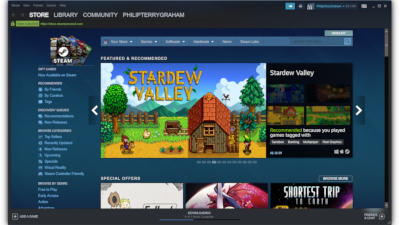This image captures the Steam interface in dark mode, characterized by a dark background and white text. The interface is divided into several sections. The upper left corner prominently features the menu options: "Store," "Library," and "Community," followed by the user's name, "Philip Terry Graham." 

On the left side of the screen, a vertical menu showcases the Steam logo at the top, with various menu options listed below in blue text against a darker blue background with white headers.

The main portion of the page is dedicated to showcasing different games available for play, with "Stardew Valley" being prominently featured. The display for "Stardew Valley" includes an animated picture illustrating a serene farm scene with a blue sky, scattered clouds, green trees, a wooden fence, and a cozy wooden cottage situated on the right side of the foreground. To the right of this image, there is a descriptor section for "Stardew Valley," including additional images and text with more detailed information about the game.

At the bottom of the screen, the "Special Offers" section is partially visible, displaying images of other offers that are available, although these images are cut off by the lower edge of the page.